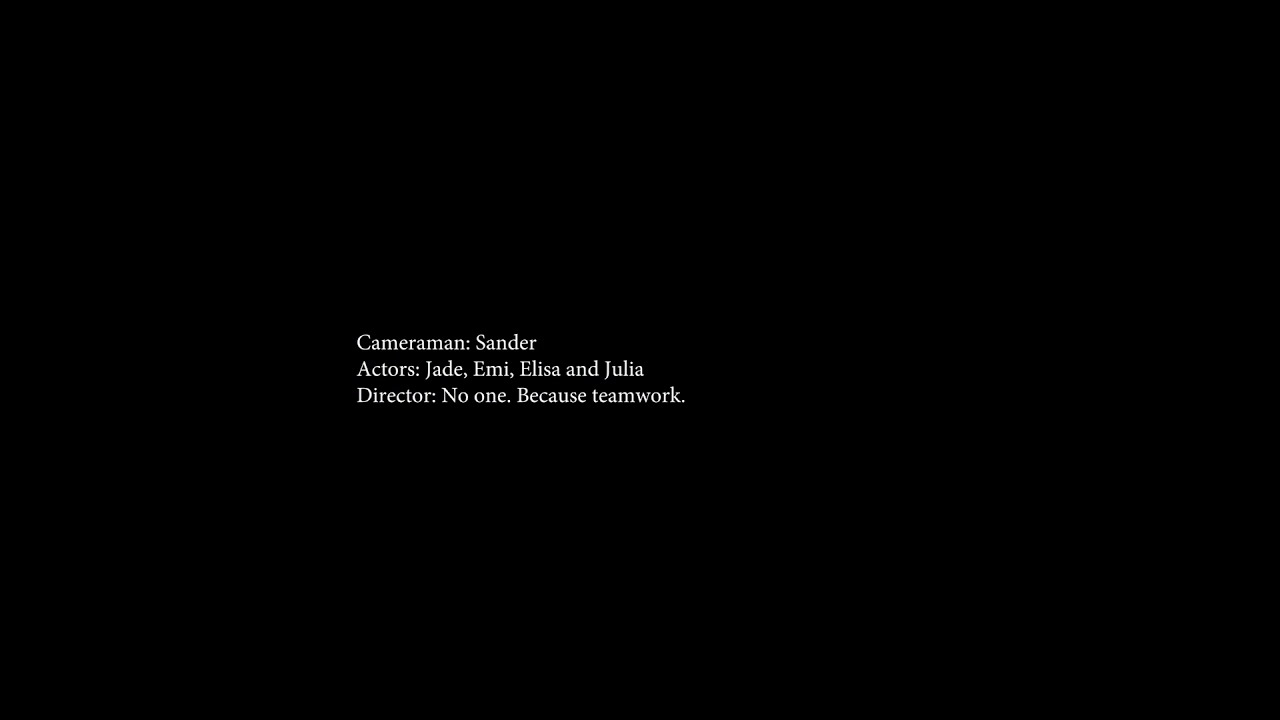The image features a landscape-oriented black background with three lines of centered white text. The font resembles a typewriter style, potentially similar to Arial or Times New Roman. The text is as follows: 

1. "Cameraman: Sander"
2. "Actors: Jade, Emmy, Elisa, and Julia"
3. "Director: no one. because teamwork."

The text is situated slightly left of the center and is relatively small, requiring closer inspection to read. This slide appears to be part of the credits for a project, emphasizing collaborative effort by noting the absence of a director.